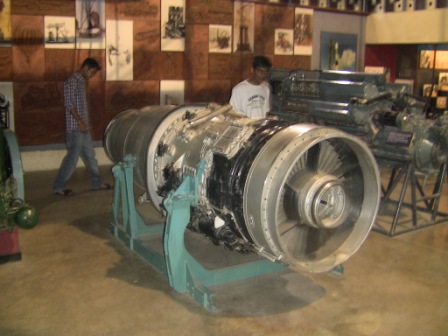The image captures an exhibit inside an aeronautics museum, featuring two large and distinct jet engines prominently displayed on elevated blue stands. The scene includes two Asian men; the one in the foreground wears a white t-shirt with indiscernible writing and has medium dark skin with short black hair, while the other, slightly behind him, sports a blue, red, and white checkered plaid shirt with sleeves rolled up to the elbows, blue Levi denim pants, and black sandals. Behind the men, to the right, there is another mechanical device, possibly another type of engine. The backdrop features a wooden-paneled wall adorned with several black and white photographs, though their details are unclear, and a screen displaying a color photo of a dog in the upper right corner. The setting and objects suggest the museum could be dedicated to aeronautics or perhaps even connected to NASA. The presence of architectural-type sketches, possibly even a space shuttle image, enhances the gallery's historical and technological ambiance.